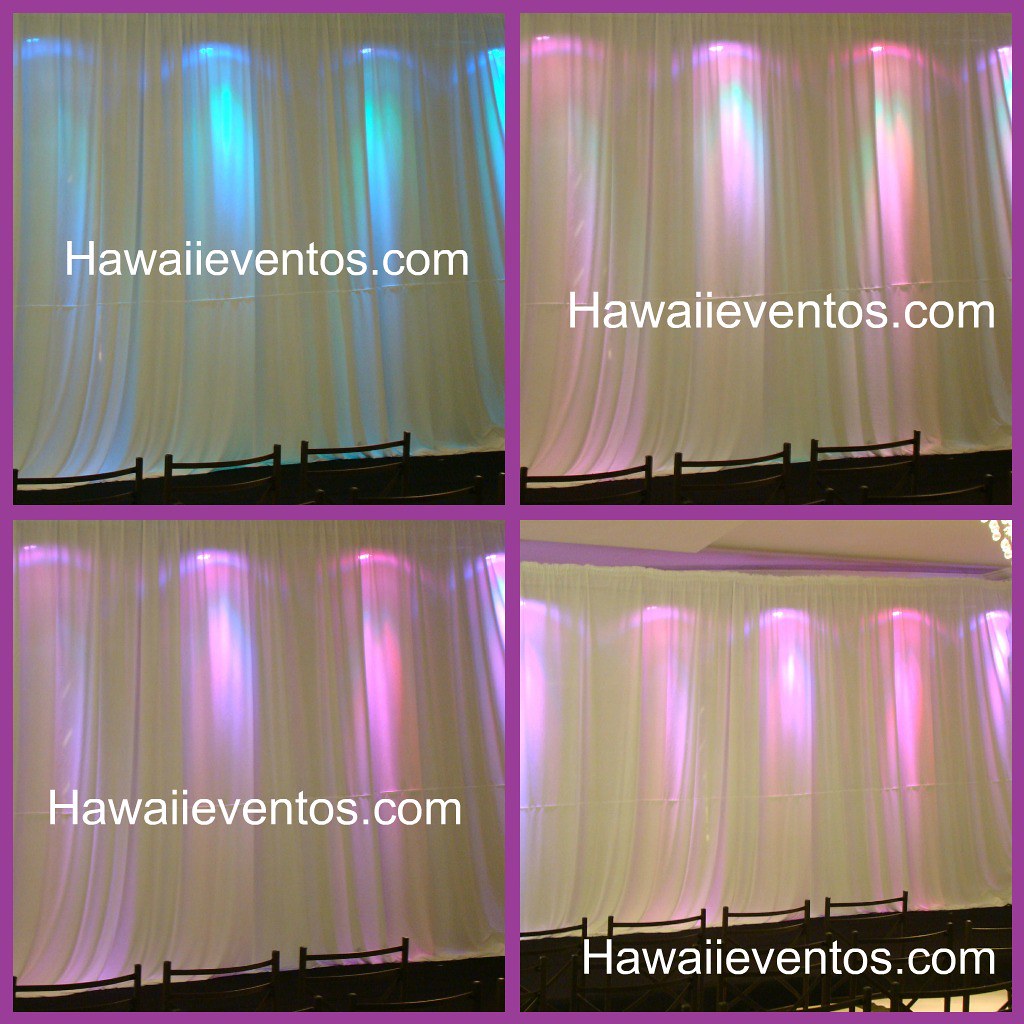The image is divided into four quadrants, each separated by a thin pink or purple border, forming a cohesive square. Each quadrant showcases a sheer white curtain with the URL "HawaiiEventos.com" written in white font. The scenes are backed by the silhouettes of three visible black chairs at the bottom of each quadrant. The upper left quadrant features deep blue lights shining through the curtain. The upper right quadrant has a mix of pink and blue lights creating a soft aurora effect. In the lower left quadrant, the lighting is predominantly purple with hints of blue. The lower right quadrant displays muted pink and purple hues. While the composition and contents are largely consistent across all quadrants, the differing light colors in each section add a unique visual dynamic to the image.